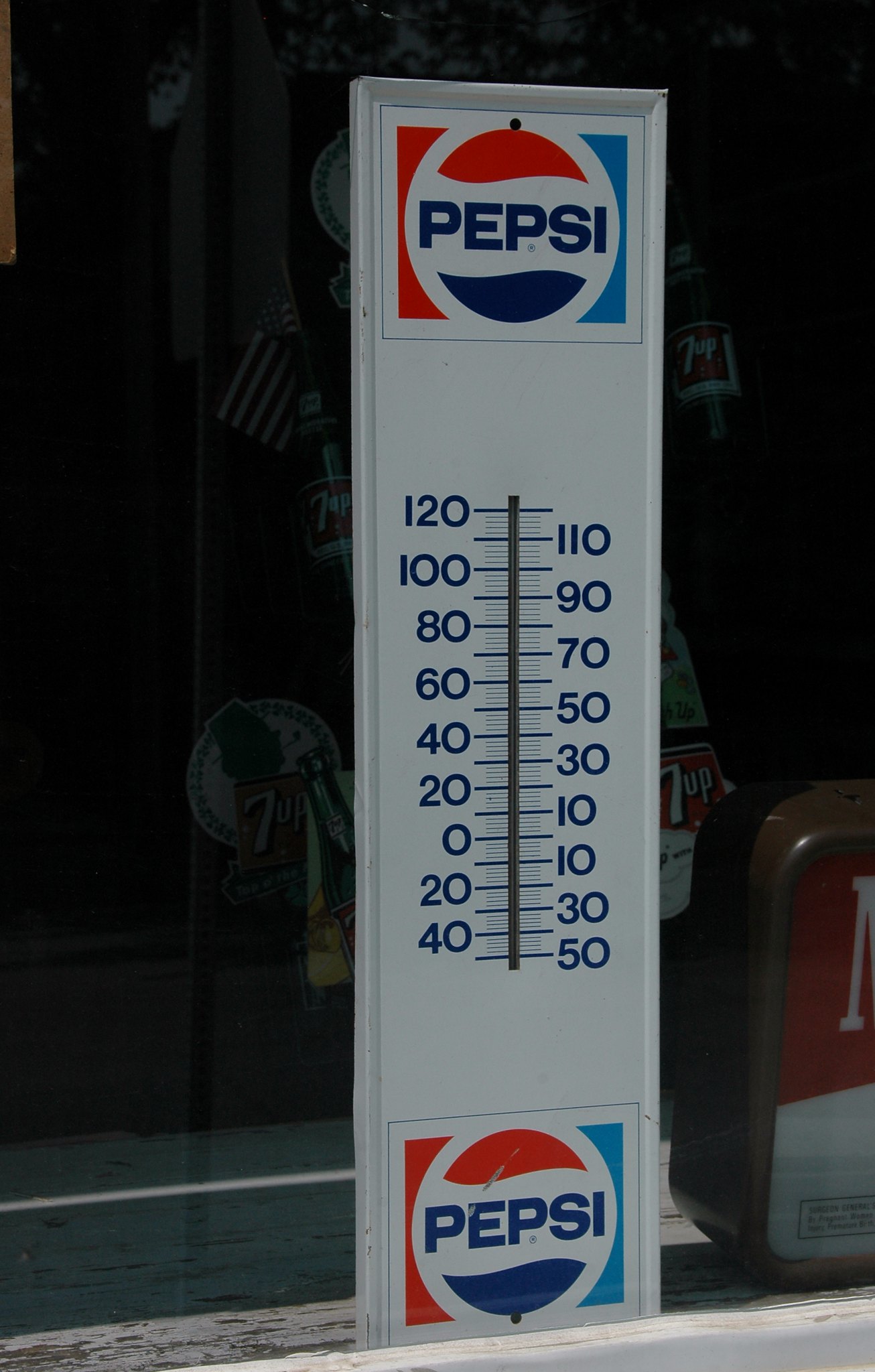A close-up vertical photograph captures a dimly lit store window. The dark background obscures much of the scene, but faint shadows reveal a collection of vintage 7up soda bottles, hinting at an American shop that might be showcasing old soda memorabilia or selling these collectibles. Dominating the center of the image is a tall, slender thermometer encased in a white box. The thermometer prominently features two Pepsi logos—one at the top and one at the bottom. The logo consists of Pepsi in large, dark blue capital letters alongside a swirly sphere, with red on the top half, dark blue on the bottom half, and a wavy white stripe cutting through the middle. The thermometer itself is vertically oriented, displaying temperature measurements from 120 to 40 degrees Fahrenheit on the left side and from 110 to 50 degrees Fahrenheit on the right side.